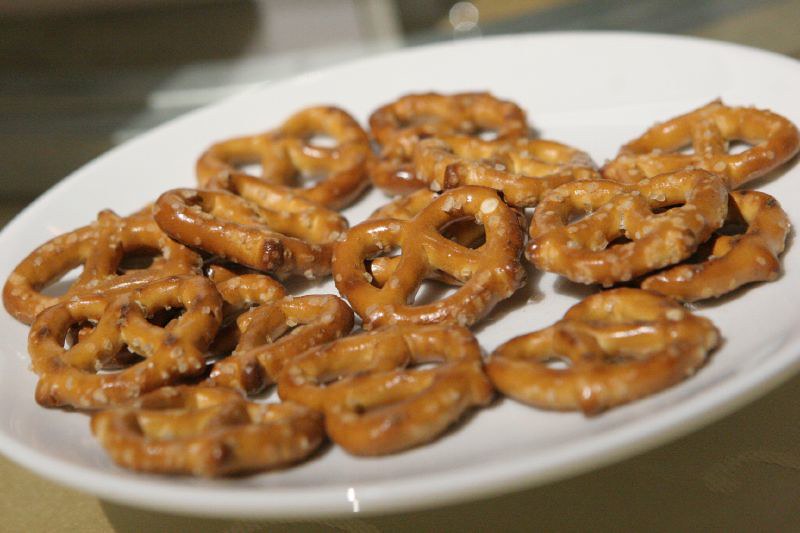This detailed photograph captures a white saucer-style plate holding approximately 20 small, hard pretzels, each twisted into a classic heart shape with their ends crisscrossed at the center. The pretzels, which are adorned with grayish salt crystals, exhibit a golden brown hue that stands out against the pristine white plate. The plate is positioned centrally in the image and is seated on what appears to be a brown table. The most prominent pretzels are those in the center, sharply in focus, while the ones toward the edges and distant background become increasingly blurry, hinting at a shallow depth of field. The overall setting suggests a casual yet meticulously arranged snack, and the composition lends an artsy touch that might indicate the photographer's interest in honing their skills. The visual contrasts of golden browns, grays, and whites create a balanced and inviting image.